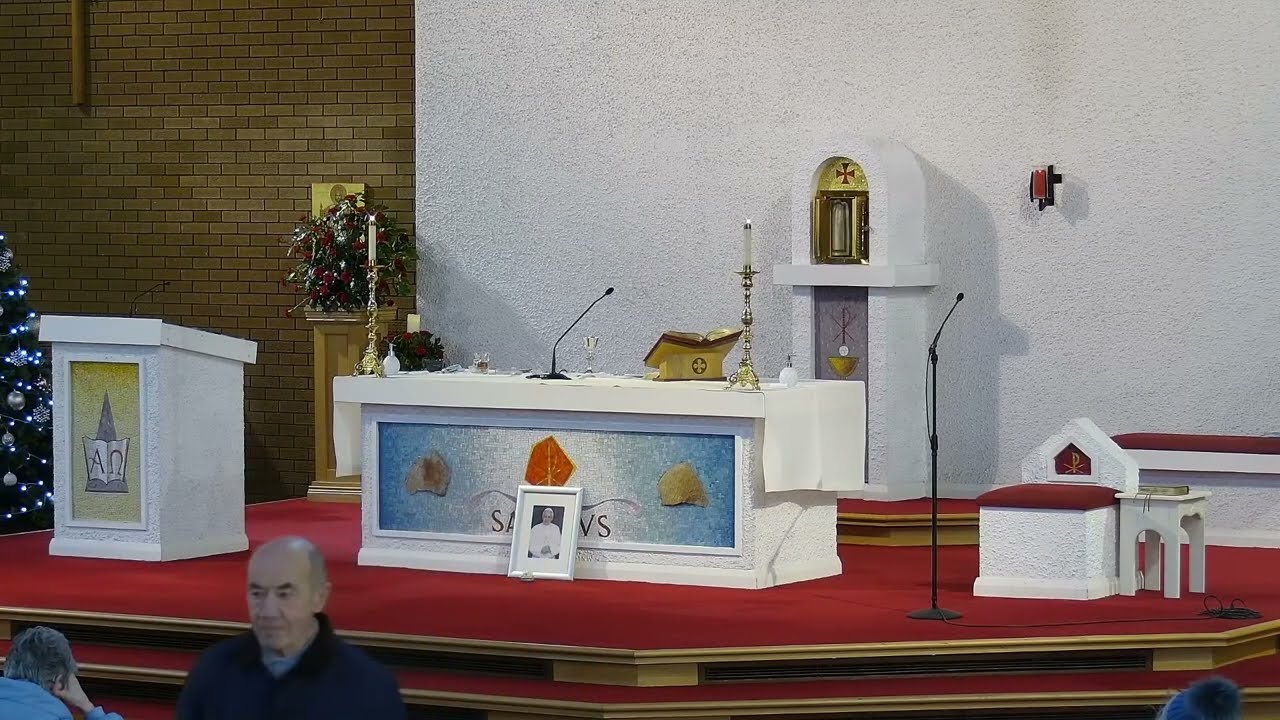The image captures the interior of a Spanish-style church, showcasing a raised platform with a vibrant red carpet. The camera is angled slightly to the right of the platform, revealing intricate details of the stage. Prominently featured on the platform is a large, white rectangular altar draped with a white cloth. Facing the altar, there is a thin microphone extending from its center. At the altar's front, there is a blue panel seemingly adorned with seashell motifs, and a photo possibly commemorating a departed priest is placed there, accompanied by a small golden stand holding a Holy Trinity Bible. 

To the left of the altar, a smaller lectern with gold artwork features a deep brown triangle design with an open Bible and an A symbol beneath an inverted horseshoe shape. Below the platform, a few congregants are visible in the foreground. Among them is an older, balding white male in a blue polo shirt, and a woman nearby with her hand clasped against her cheek.

The stage is flanked by steps with light wood trim leading up to it. On the far left, behind a dark brown brick wall adjoining a white wall, a Christmas tree adorned with white lights and silver ornaments signals the festive season. To the right of the altar, the platform also holds a small cushioned red chair, a candlestick, and an end table or coffee table with a book on top. The backdrop of the scene is a pristine white wall, enhancing the church's serene and holy ambiance.